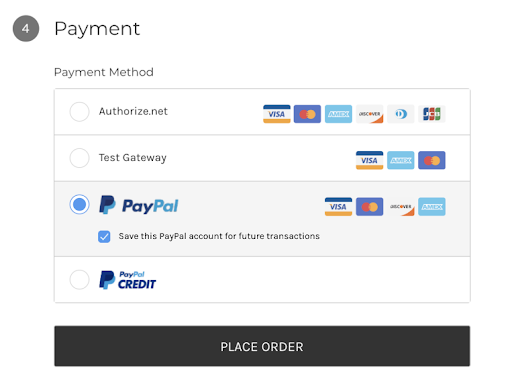The image depicts a website's payment page. At the top of the page, there is a grey circle with the number "4" inside, accompanied by the heading "Payment" in black text. Directly beneath this, the page displays "Payment Method" and offers four distinct options:

1. **Authorize.net:** This option includes a variety of icons representing different credit card providers—Visa, MasterCard, American Express (Amex), Discover, a card with a "D" in the center on a blue and white background, and JCB.
2. **Test Gateway:** This option shows icons for Visa, Amex, and MasterCard.
3. **PayPal:** Featuring the PayPal logo with two overlapping "P"s (one darker blue, the other lighter blue), this option includes icons for Visa, MasterCard, Discover, and Amex. A checkbox next to this option is selected, with the text "Save this PayPal account for future transactions" displayed on a blue background.
4. **PayPal Credit:** This option includes the PayPal logo and the words "PayPal Credit" in blue.

At the bottom of the page, there is a "Place Order" button, which has white text on a black background indicating it is the final step to complete the purchase. The overall layout of the page features a white background with black text.